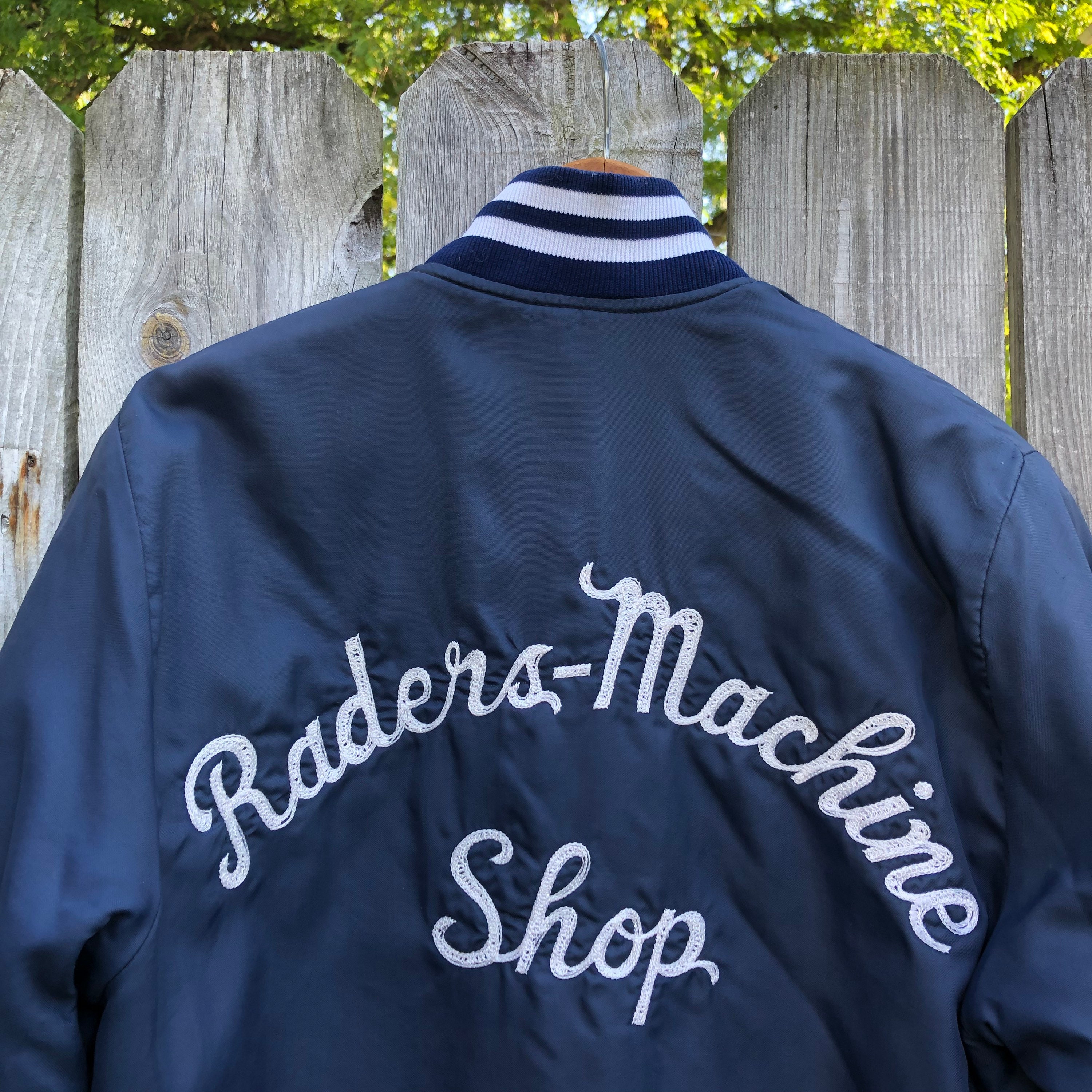This outdoor daytime photograph showcases a work jacket hanging on a weathered gray wooden fence. The jacket, slightly wrinkled and hung on a silver metal hanger, is dark blue with a bit of shine. It's adorned with a stretchy collar featuring horizontal stripes in dark navy and white. In white cursive lettering across the back, the text reads "Raiders Machine Shop." The upper part of the image features some out-of-focus green and slightly yellowing leaves, hinting at a backyard setting. The image appears to be a simple, possibly amateurish product photo, potentially for an online listing such as eBay. The colors in the image are predominantly blue, white, light wood, and green, emphasizing the casual and unrefined nature of the photograph.